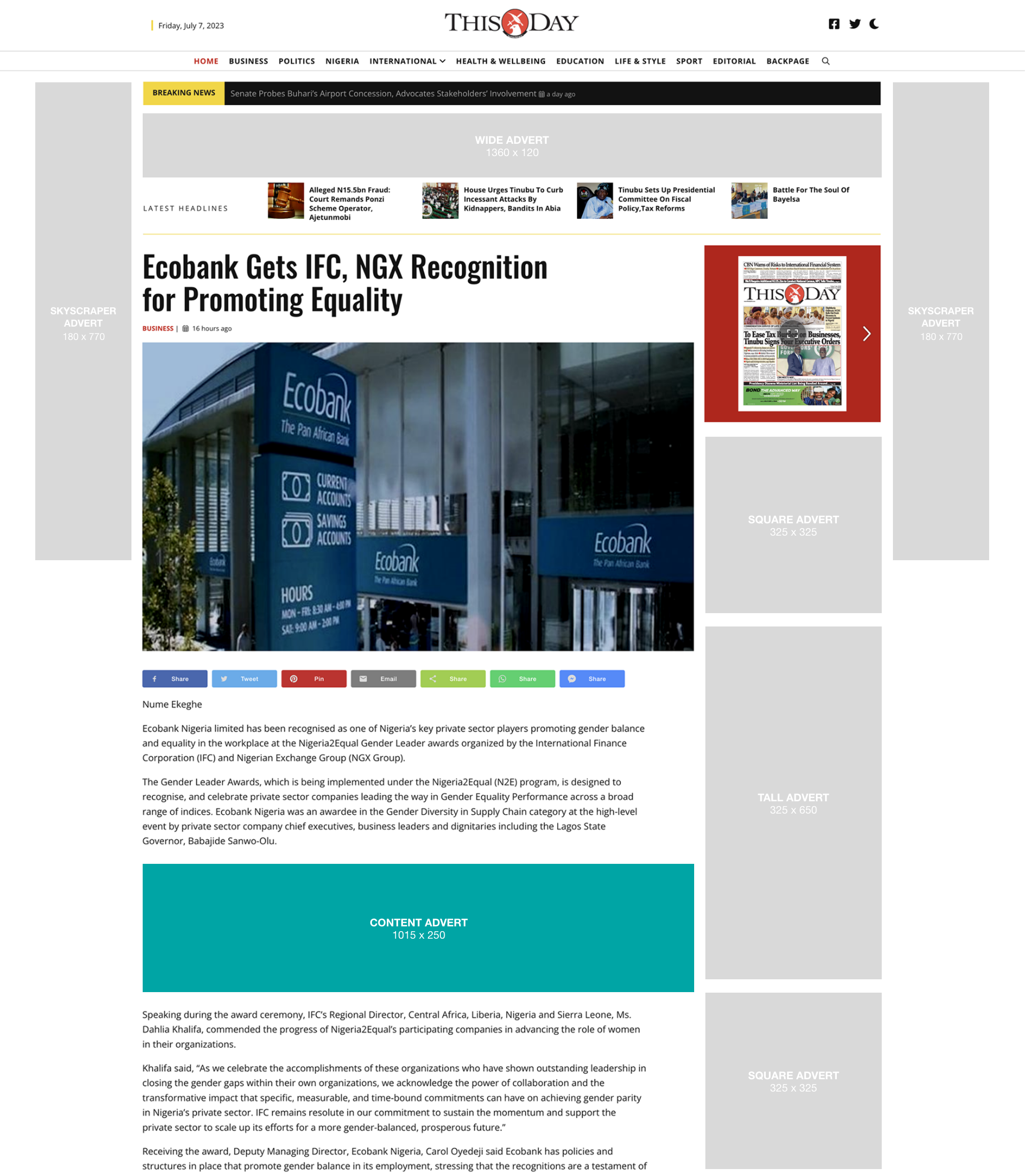The image portrays a detailed snapshot of a news website's homepage. At the very top, there is a clean, white header featuring a slender yellow line. It prominently displays the date, "Friday, July 7th, 2023," alongside the caption "This Day" in capitalized letters. Between the words "This" and "Day," there is a distinct round red circle edged in black, containing an image of a bird with an X over it.

To the right of the header, icons for Facebook, Twitter, and a crescent moon are visible, likely representing links to social media and a toggle for a dark mode feature. Below the main header, a navigation bar lists various sections of the website, starting with "Home" highlighted in red, followed by sections such as Business, Politics, Nigeria, International with a dropdown menu, Health and Wellbeing, Education, Life and Style, Sport, Editorial, and Backpage. A magnifying glass icon indicates the search function for the site.

Further down, a bright yellow banner announces breaking news in capitalized black text. Just below, a black background with white text reads, "Senate probes, Ferraris, Airport concession, Advocates, and Stakeholder Involvement."

Continuing down the page, there's a gray banner marked "White Advert," followed by a section on a white background labeled "Latest Headlines," listing the most recent news stories. Dominating the main page is a headline: "Echobank gets IFC, NGX recognition for promoting equality," accompanied by an image of Echobank. Adjacent to the main article, the right sidebar displays multiple advertisements and banner slots available for purchase, enhancing the page's commercial aspect.